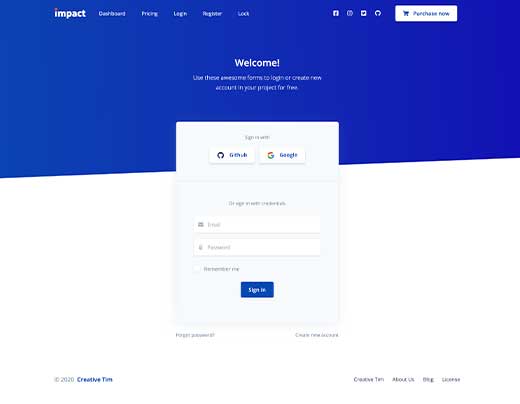The image depicts a web page, specifically a login page for a website named "Impact," identifiable by the word "Impact" with a red dot above the lowercase 'i'. The page has several key sections and features, starting with a blue bar at the top that includes a welcoming message and possibly the phrase "awesome forms" which could be the site's tagline. 

In the upper right-hand corner, there is a white button labeled "Purchase Now" with a shopping cart icon next to it. The site’s main navigation menu includes links to "Dashboard", "Pricing", "Login", and "Register". 

Below the blue bar, there is a login form consisting of fields to input an email address and password, along with a "Remember me" checkbox. The "Sign In" button, styled in dark navy blue with white lettering, is prominently placed. There is also a "Forgot Password?" option on the bottom left of the login form, as well as a "Create Account" option on the other side.

At the bottom left of the page, the footer displays the text "2020 Creative [something]", indicating the possible copyright or creator's information, while the bottom right contains a series of smaller menu items. The overall design and functionality suggest it is a standard login page, though the poor resolution makes reading some parts difficult.